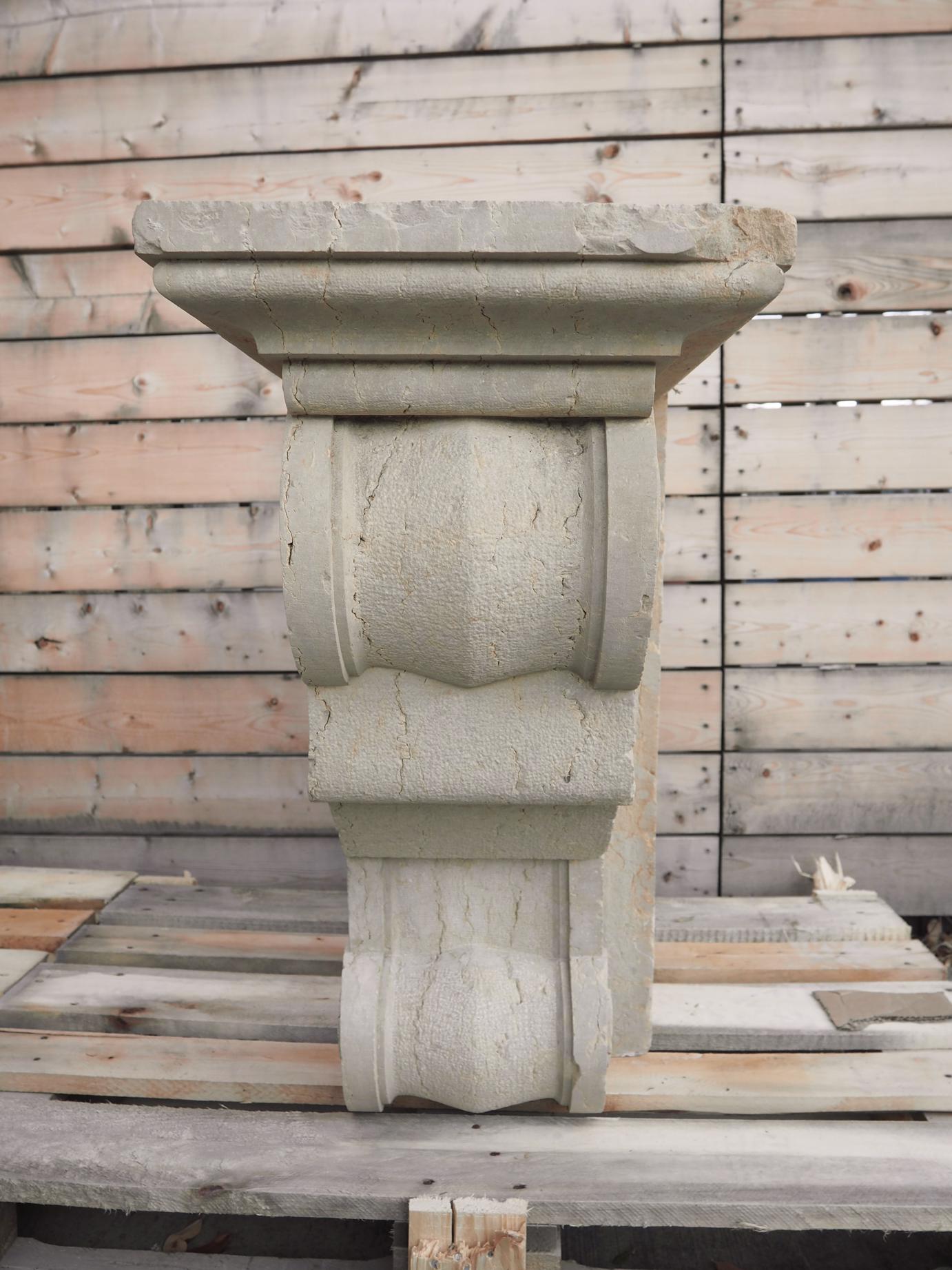This photograph captures a richly textured scene featuring a rustic composition of wood and stone. Dominating the foreground is a large, heavy-looking concrete statue resembling a pedestal, characterized by its rough surface with prominent chips, crags, and cracks. The pedestal, whitish in color, tapers from a narrower bottom up to a broader square tabletop. Nestled atop a set of horizontal wooden slats that form both the floor and the backdrop of the image, the wood elements display a range of natural hues from off-white, beige, and tan to grayish tones. The wooden planks are visibly nailed together, presenting a raw, rustic aesthetic with noticeable gaps and cracks that allow glimpses through the wall. This detailed interplay of diverse textures and colors creates a striking contrast between the organic, weathered wood and the imposing, sculpted stone centerpiece.